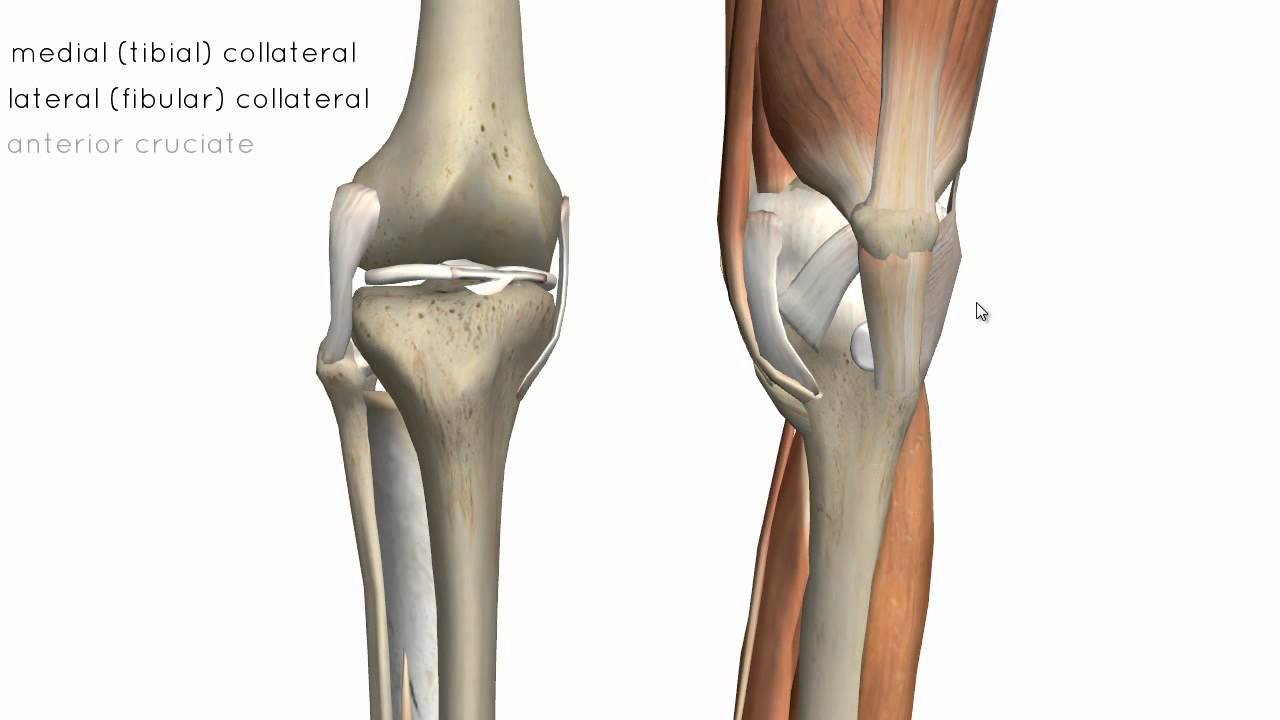The image is a detailed, computer-generated diagram of the human knee joint, presented against a white background. On the left side of the image, there are three lines of text. The top two lines, inscribed in black, read "medial (tibial collateral)" and "lateral (fibular collateral)." The third line, in a lighter gray color, reads "anterior cruciate."

The diagram consists of two separate images side by side. The left image provides a straight-on view of the knee joint, showcasing the femur (upper bone) and the tibia and fibula (lower bones) in a realistic, grayish-silver color. Tendons connecting the bones are shown in white, and there is a thin layer of cartilage visible between them. The right image presents a side view of the same knee joint, but this time with surrounding muscles depicted in light brown. This side view highlights the detailed connections between the bones, tendons, and muscles, offering a comprehensive understanding of the knee joint's anatomy. Though the illustrations are not highly detailed, they provide clear, 3D-like visualizations of the knee structures.